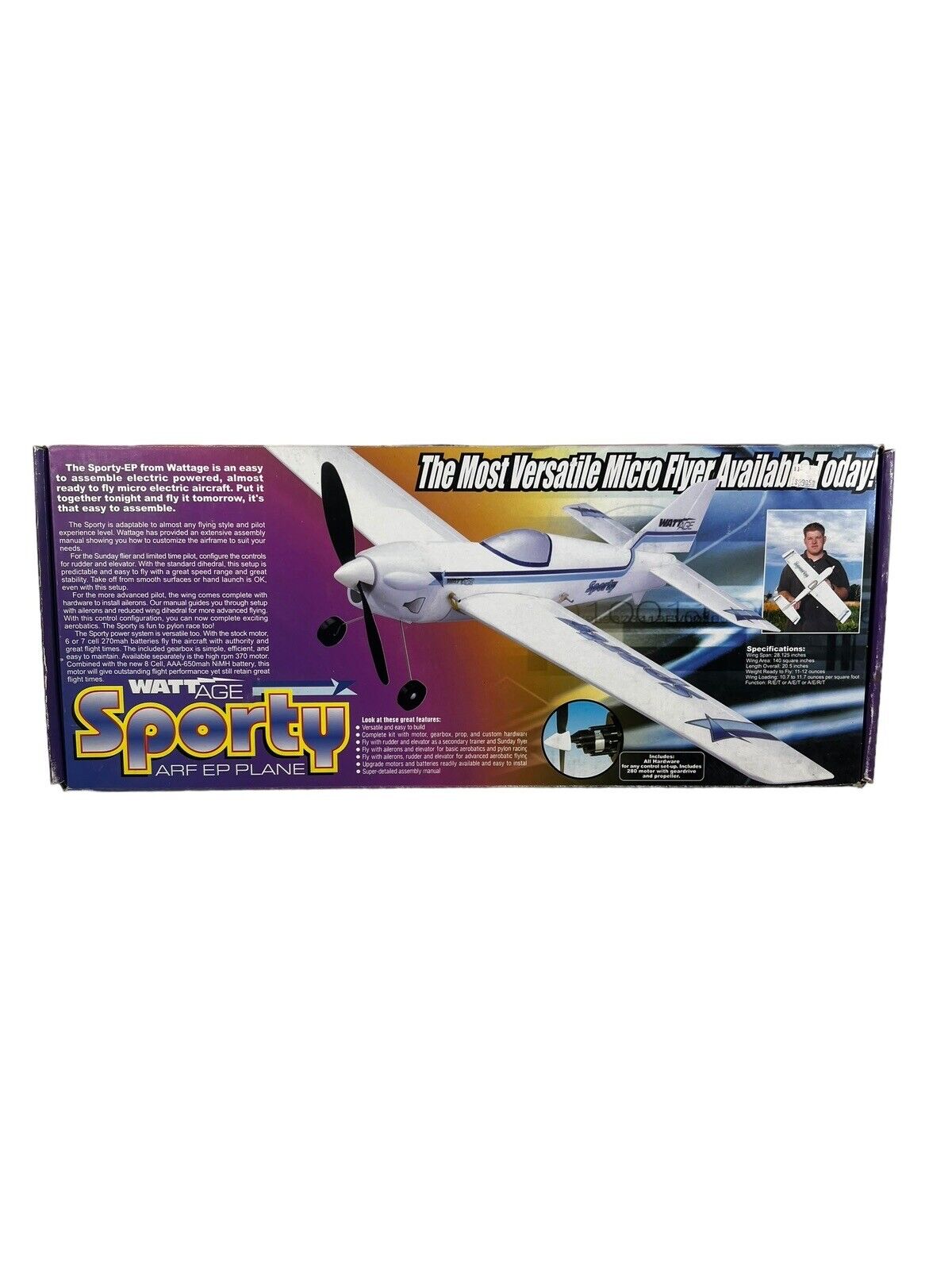The image shows a package for the "Wattage Sporty ARF EP Plane," a detailed remote control micro flyer, touted as the most versatile available today. The sleek airplane is all white with distinctive black and light blue stripes running down its center body and along its wings. The packaging features a photograph of a man holding the aircraft, illustrating its compact size, roughly extending to the man's chest. The plane includes two black wheels for easy landing. Notably, the box highlights the plane's ease of assembly, emphasizing that it can be put together tonight and flown the next day. The top left corner of the package offers a description of the airplane as an "easy to assemble electric powered, almost ready to fly micro electric aircraft." Additionally, the box displays specifications, including wingspan, wing area, length, and overall weight, though some text is difficult to read.